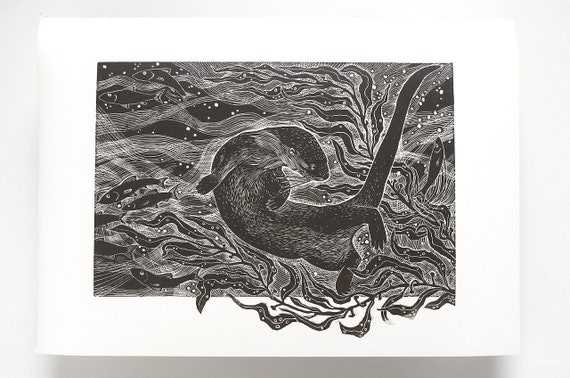This is a detailed black and white illustration of a sea otter swimming in the water. The otter’s body is dynamically twisted, with its lower half positioned horizontally and its upper body turning vertically to the right, creating a sense of movement as it swims among the underwater currents. The tail of the otter extends to the right side, while its head is angled down towards the bottom right corner of the image. Around the otter, artistically drawn wavy white lines depict the water currents flowing from right to left, interspersed with bubbles. The scene includes sea kelp originating from the bottom right corner and flowing to the left, wrapping around part of the otter. The image also features several black fish: three in the bottom left corner swimming to the left, two at the top left also going left, and one on the right side swimming upwards. The intricate shading in black, grays, and off-whites enhances the depth and texture of the underwater environment.